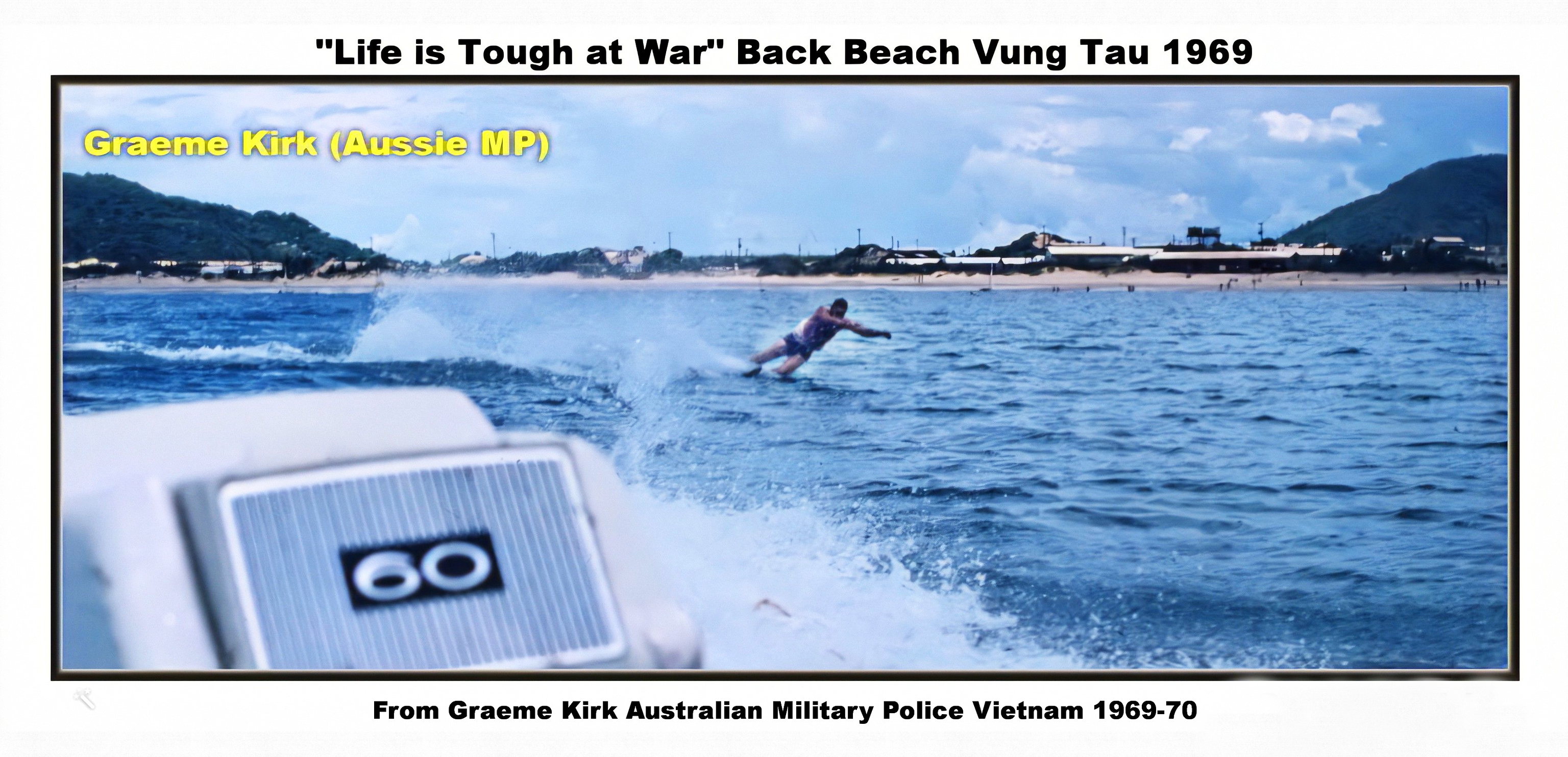This wide-angle color photograph, taken from the perspective of a motorboat in calm waters, captures a moment at Back Beach, Vung Tau, Vietnam, in 1969. The image highlights a water skier gliding on blue waters behind the boat. Above the photo, yellow text reads "Life is Tough at War," while additional captions identify the scene: "Back Beach, Vung Tau, 1969" and "From Gramey Kirk, Australian Military Police, Vietnam, 1969 to 1970." The text at the top left corner mentions "Gramey Kirk, Aussie MP." In the background, a shoreline dotted with buildings and a tree line suggests a military base, and distant figures can be seen on the beach.